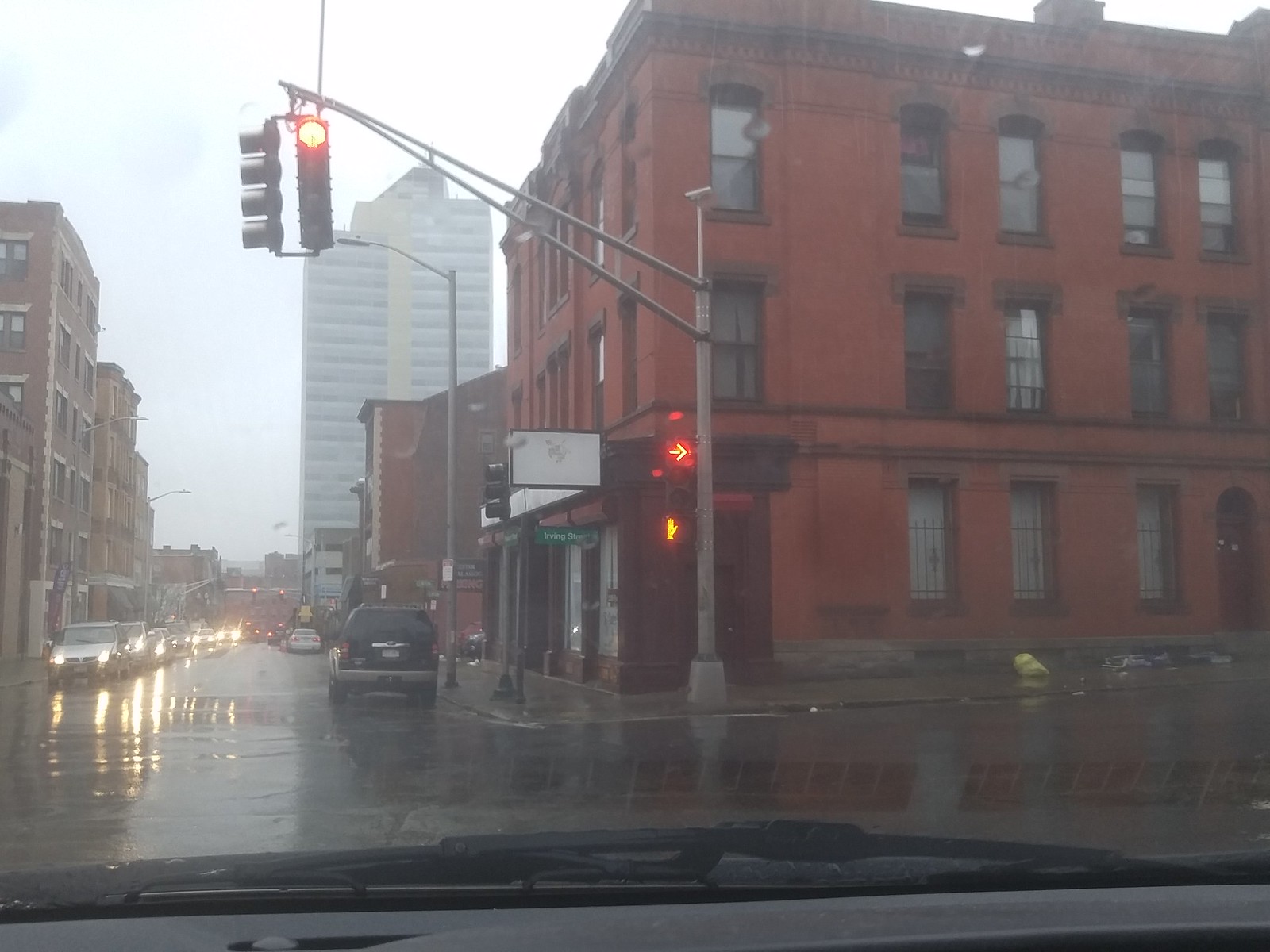The photograph captures a rainy city street from inside a car positioned at a red traffic light. The black dashboard and stationary windshield wipers are visible through the windshield. To the left, there are tall, brownish brick apartment buildings, one boasting six floors with two windows per floor. A large white building, likely corporate or office space, looms further in the background. On the right side of the image, a three-story red brick building with barred windows is prominently featured. The car appears to be in the right lane, waiting to turn right, with a red right-turn arrow visible. Across the street, oncoming traffic is also halted at the red light, with numerous cars' headlights reflecting on the wet roadway. The street additionally showcases parallel-parked cars, primarily on the right. Overall, the scene illustrates the gritty yet captivating atmosphere of a city in the rain, with a blend of residential and commercial architecture framing the view.